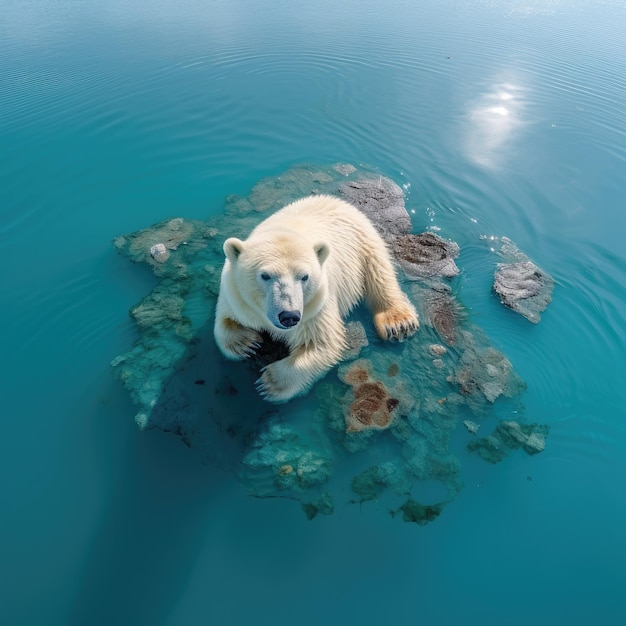A stunning aerial close-up captures a majestic polar bear resting on a small, coral-like island. The bear, with its white fur tinged slightly yellow, looks up towards the camera, though its gaze is directed slightly downward. From this overhead perspective, both the top of the bear's head and much of its back are visible. The tiny piece of land it sits on is surrounded by water, which dominates the majority of the image and accentuates the isolation and vulnerability of the scene. The vivid contrast between the bear's pale fur and the deep, encompassing water makes the polar bear the undeniable focal point of this poignant photograph.